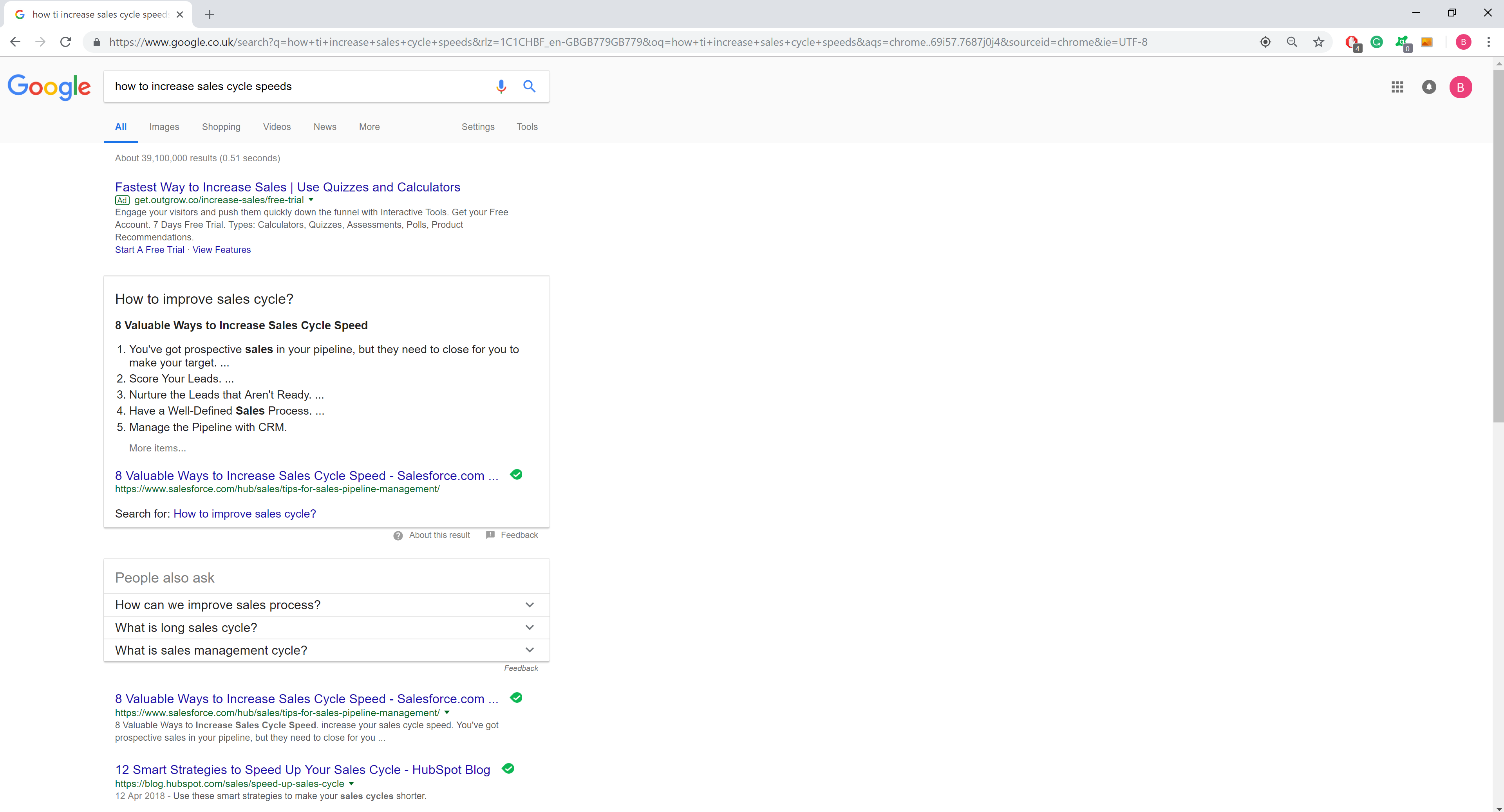A screenshot of a desktop displaying the Opera browser with a single tab open to a Google.co.uk search. The browser window is unusually configured, occupying only the left 30% of the screen. At the top left, below the URL bar and navigation buttons, is the prominent Google logo. The user has searched for "how to increase sales cycle speeds." The first result is an advertisement titled "Fastest Way to Increase Sales," followed by a Google info box outlining five methods to improve sales cycles. Below this info box is a "People also ask" section, and further down are actual website results related to the search query.